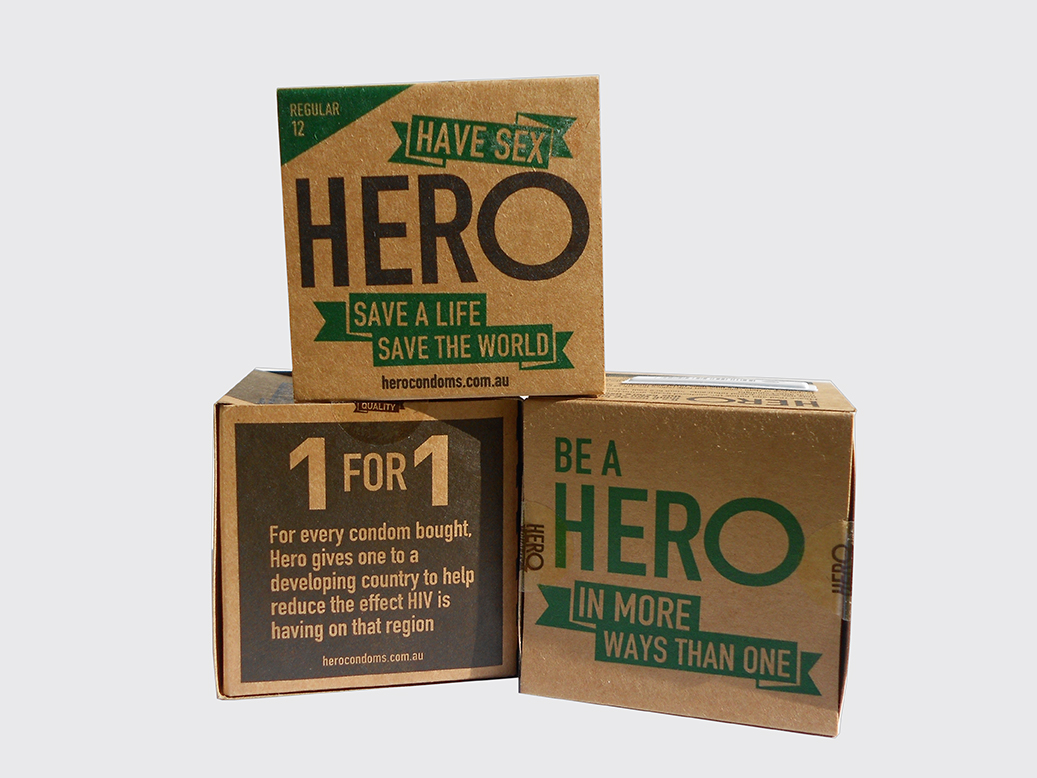The image displays three brown packages of Hero Condoms against a clean, gray background. Each box is labeled with "Regular 12" in green at the top corner. Prominently featured text on the boxes says, "Have sex, hero. Save a life. Save the world." The packaging highlights the brand's mission at herocondoms.com.au, stating that "For every condom bought, Hero gives one to a developing country to help reduce the effect HIV is having on that region." Additionally, a message on the bottom right of the packaging reads, "Be a hero in more ways than one." Each package is a small square box, and the arrangement in the image has two boxes at the bottom with one stacked on top.